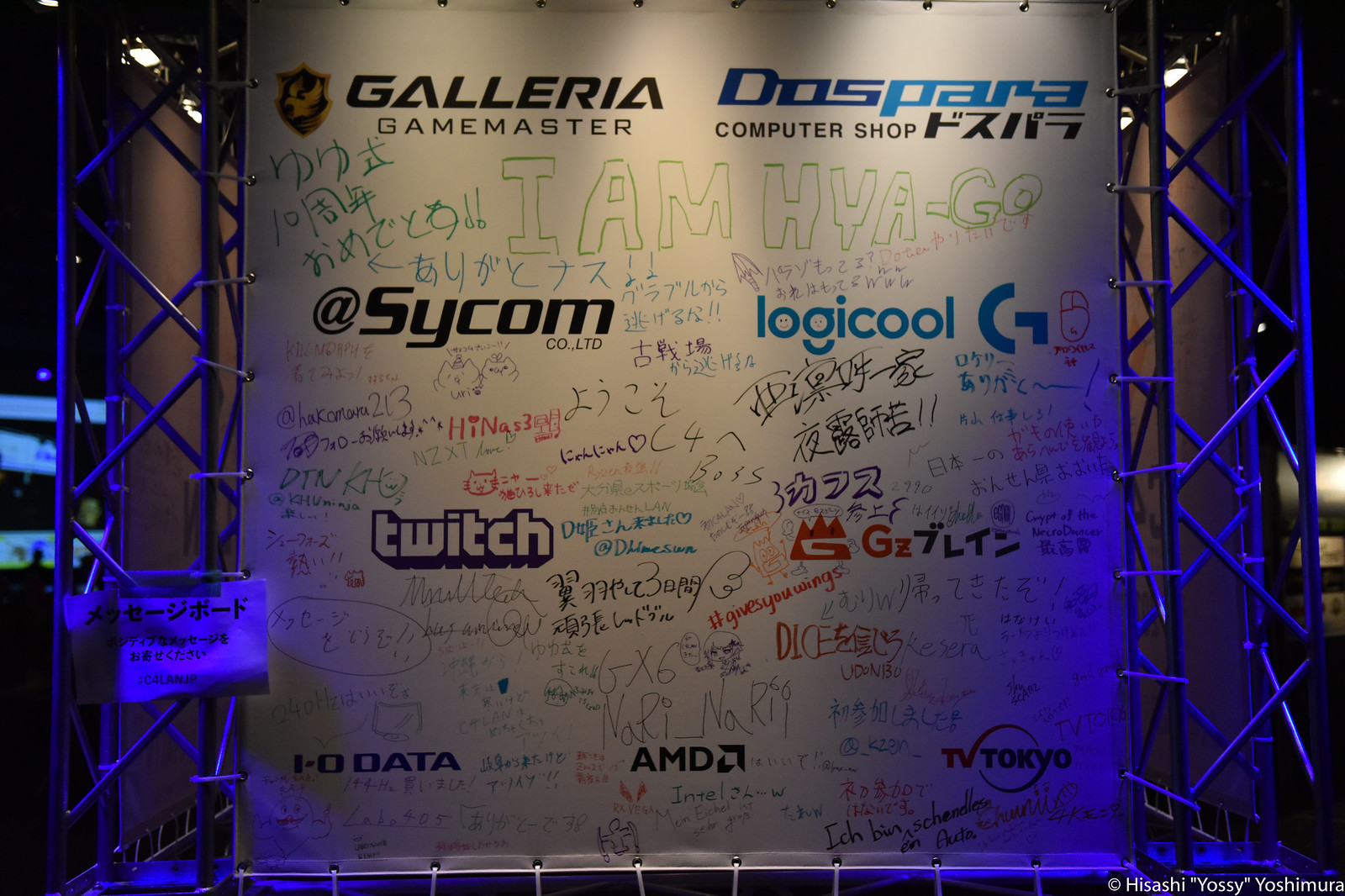This detailed color photograph, captured in landscape orientation, showcases a section of wall entirely filled with various computer-related brand names, such as AMD, SICOM, Twitch, Logicool, Dospara's, Galleria, and Gamester, hinting at a possible gaming conference setting. The wall, which resembles a whiteboard or greaseboard and occupies the full height and most of the width of the image, is adorned with handwritten signatures and multicolored marker text, primarily in black, blue, and green. Flanking either side of this central display are metal frames, secured to the sign with zip ties. Accentuating the scene, blue-hued light highlights the edges of the frames and portions of the sign itself, while scaffolding, potentially purple due to the lighting, forms part of the backdrop. The photograph, a realistic interior shot, expertly combines graphic design elements with the spontaneous style of personal signatures, set within an environment suggestive of a tech or gaming event.